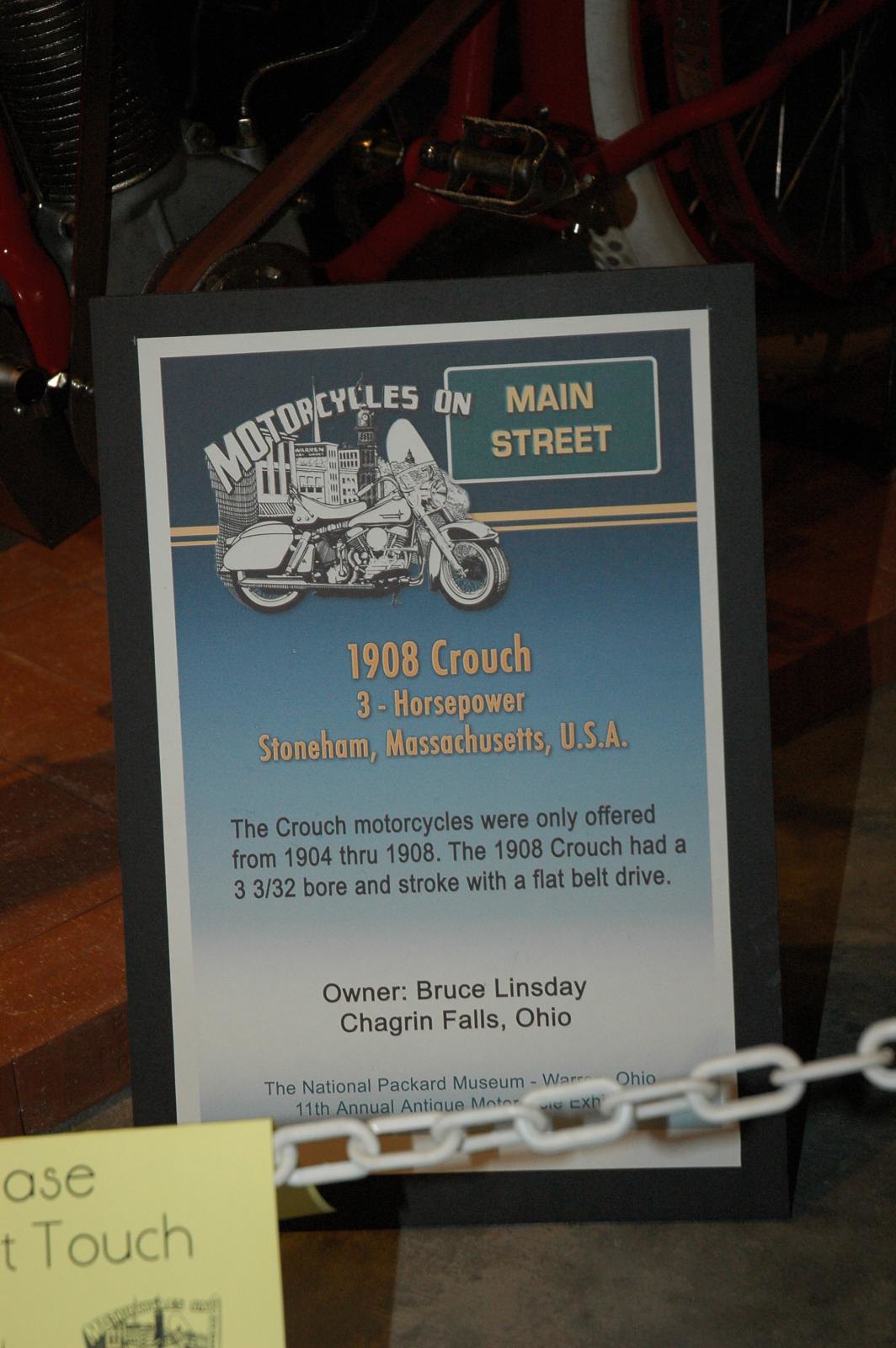This color photograph captures a centrally placed, intricately detailed sign with a black and white border. The background of the sign transitions from dark blue at the top to white at the bottom, producing a gradient effect.

At the top of the sign, there is a vintage black and white image of a motorcycle oriented towards the right. Immediately above this image, in white lettering, is the text "Motorcycles On." To the right of the motorcycle image is a green street sign with yellow lettering that reads "Main Street," highlighting the shop's name, "Motorcycles On Main Street."

Beneath these elements, prominently displayed in yellow text, the sign reads: "1908 Crouch, 3 horsepower, Stoneham, Massachusetts, USA." Below this, in black text, additional information about the motorcycle is provided: "The Crouch motorcycles were only offered from 1904 through 1908. The 1908 Crouch had a 3 3/32 bore and stroke with a flat belt drive." At the very bottom of the sign, also in black text, is the owner's information: "Owner Bruce Lindsay, Chagrin Falls, Ohio."

In front of the sign, there is a white chain with a yellow sticky note attached to it, displaying the partial word "touch" in black lettering. Behind the sign, a red bicycle is faintly visible, adding another layer of interest to the scene.